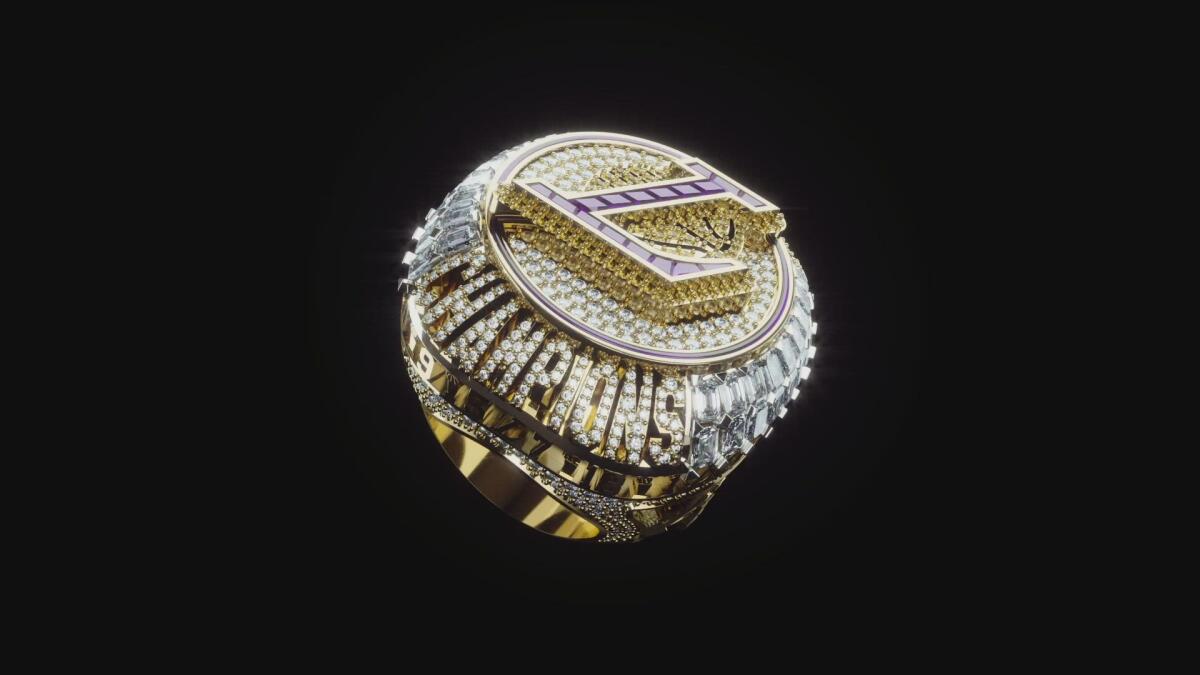This image showcases an exquisite championship ring, likely from a prestigious football or sports event. The ring is predominantly gold, adorned with countless diamonds, which give it an opulent sparkle. At the center of the ring sits a prominent letter "L," featuring a purple backdrop, symbolizing victory or a team’s initial. The "L" is encircled by a gleaming gold ring, itself encrusted with further diamonds that enhance its magnificence. The base of the "L" is crafted in gold, adding to the luxurious details.

Below this central emblem, the word "CHAMPIONS" is meticulously spelled out in diamonds, emphasizing the ring's significance. Flanking this word are larger diamonds that run along the sides of the ring, adding to its grandeur. The lower portion of the ring showcases a gold area, adorned with a diamond-shaped pattern, creating an intricate and cohesive design. All of these elements come together on a striking black background, making the ring's details even more vivid and dazzling.